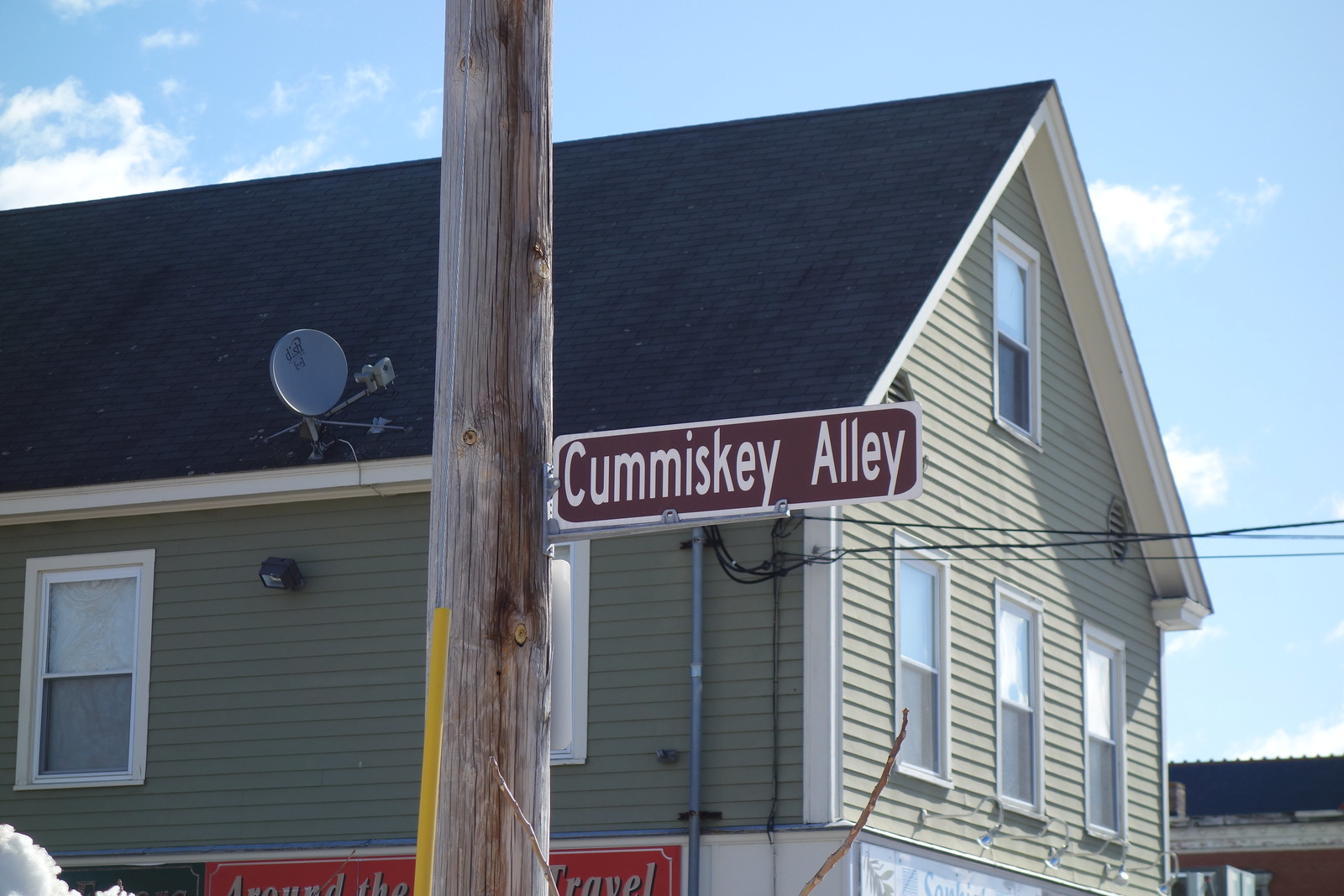This photo, taken outdoors on a sunny day, captures a residential scene featuring a prominent wooden utility pole in the foreground. The pole, tall and made of brown wood, supports several black wires and is marked with a brown street sign bordered in white, reading "Comiskey Alley."

In the background stands a two-story house with light green vinyl siding and an A-frame roof covered in black shingles. The house is outfitted with a small, gray satellite dish mounted on the side. Visible on the house are three evenly spaced windows on the lower floor and one window on the upper floor, along with two windows on the side facing the camera. There's an obscured sign on the house with partially readable text, including the words "around the travel." Additionally, a black square light fixture is attached to the side of the house.

The sky above is a clear blue with a few scattered white clouds, further enhancing the outdoor setting. In the lower right corner of the image, another house is visible in the distance, identifiable by its black roof.